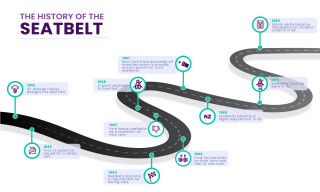The image displays an intriguing infographic on a white background that traces the history of the seatbelt. At the top, in purple text, it prominently states "THE HISTORY OF THE SEATBELT". The central feature is a winding, serpentine roadway that curves from the left to the right, symbolizing the timeline of seatbelt development. Along the road are numerous turquoise pointers and light blue circles with small icons that mark significant milestones in the history of the seatbelt. Each point is accompanied by a text box offering detailed information, but unfortunately, the text is extremely small, blurry, and difficult to decipher, even with the use of a magnifying glass. The combination of these elements visually narrates the evolution and extensive testing and changes of the seatbelt over time, although the specifics are frustratingly illegible.